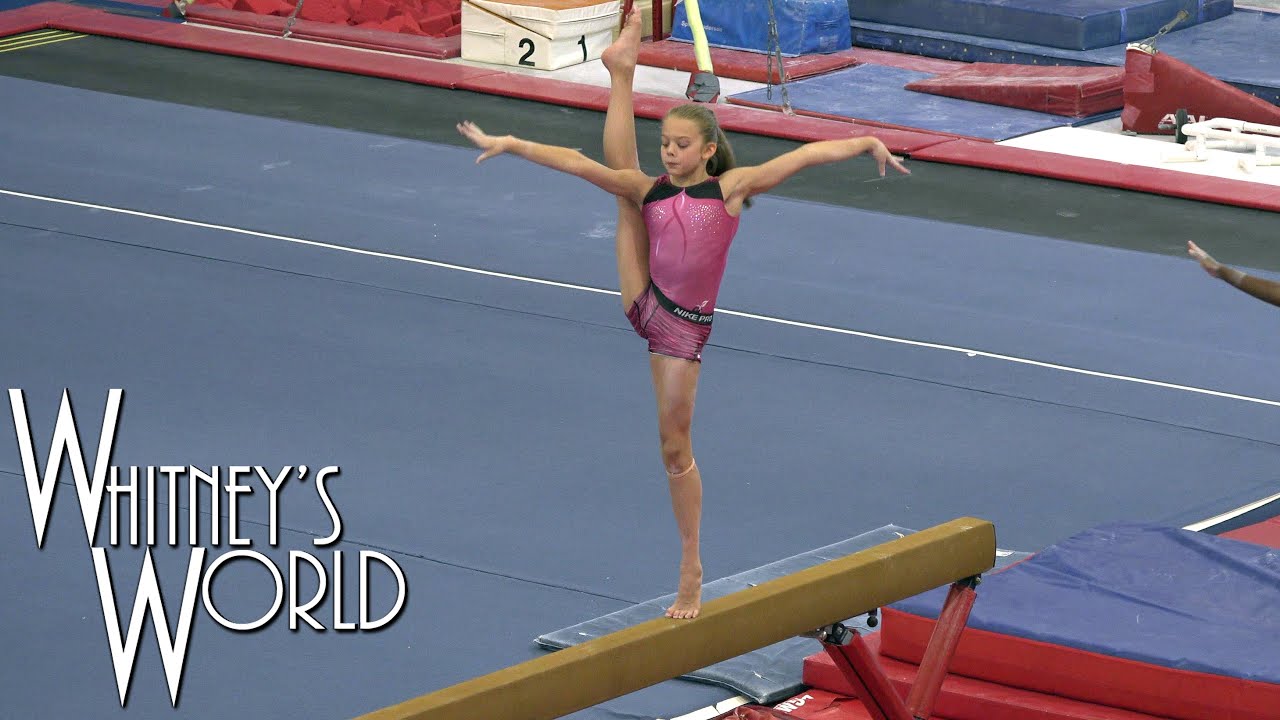The photograph captures a young gymnast skillfully performing on a wooden balance beam in what appears to be a gym setting. The gymnast is dressed in a pink jumpsuit with a black border at the top and a black Nike belt. She maintains her balance with both arms extended, one hand flaring down and the other up, while one leg is firmly planted on the beam and the other is lifted high into a split-leg position. Positioned on the beam's surface are two red foam X's at either end, and several blue and red mats are scattered around the area, indicating a well-padded environment typical of gymnastic meets. The gym floor, marked with white lines, adds to the authentic gym atmosphere. On the bottom left corner of the image, the text "Whitney's World" is prominently displayed in large white font. In the background, only the arm of another gymnast can be seen, highlighting the girl's focused performance amid a busy gym scene.